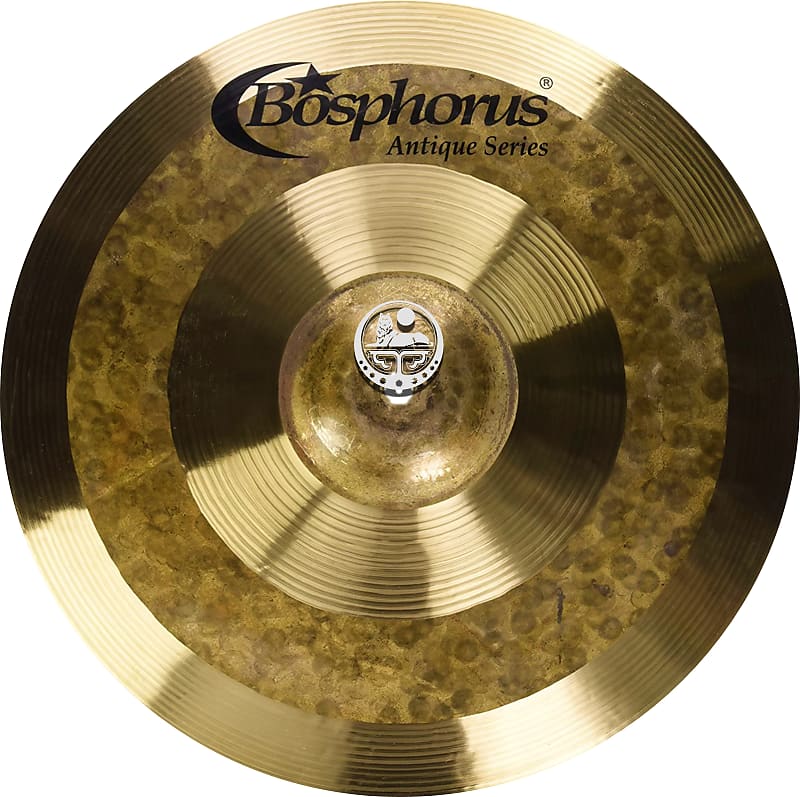In this image, we have what appears to be a cymbal from the Bosphorus Antique Series, distinguished by its circular, shield-like design. The cymbal has a striking appearance with a predominantly gold surface that alternates between smooth and mottled textures, reminiscent of a dirty, spotted yellow in some areas. Around the outer edge, the cymbal maintains a clean gold finish, but transitions into a spotted texture towards the center, creating a layered effect. In the very center, there's a silver emblem which might be a small coat of arms featuring what looks like a lion or wolf lying down—a detail too small to identify with certainty. Above this emblem is a distinctive logo with black text spelling "Bosphorus Antique Series," accompanied by a crescent moon and star over the 'O', adding an ornate touch. The cymbal's metallic sheen catches the light brilliantly, enhancing its antique allure.